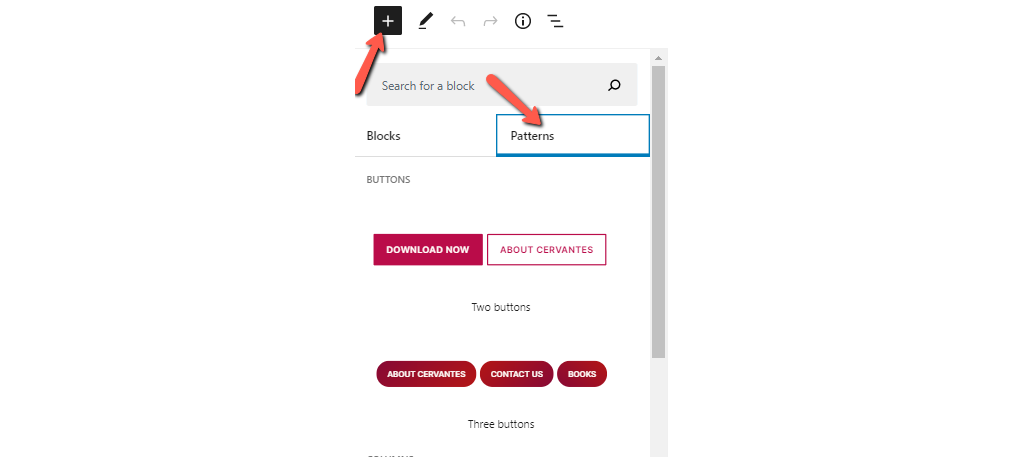This screenshot appears to be from a web or mobile-based editor, potentially used for designing or customizing a website or blog. The interface includes multiple highlighted elements, marked by bold light orange-red arrows and a blue rectangle for emphasis. 

At the top of the screen, there is a white plus icon inside a dark gray square, next to which is a light orange-red arrow. Adjacent to this are several icons lined up in sequence: an edit pencil, back and forward navigation buttons, an information (info) button, and a unique icon consisting of three staggered, stacked lines. Below this row of icons, there is a search bar accompanied by a magnifying glass icon labeled "Search for a block." 

Next to the block search bar are two options: "Blocks" and "Patterns." The "Patterns" option is highlighted by both a light orange-red arrow and circled with a blue rectangle, drawing attention to this particular feature. Below this highlighted section, labeled "Buttons," there are two button options. On the left, a solid magenta button reads "Download Now" in white text. To the right, an outlined white button with magenta text reads "About Cervantes."

Beneath these buttons, the caption specifies another section labeled "Two buttons," featuring three pill-shaped buttons: "About Cervantes," "Contact Us," and "Books," all with white text on a burgundy background. Below this "Two buttons" section, there's a "Three buttons" label reinforcing the count of buttons displayed. Finally, a light gray scroll bar runs along the right side of the interface, indicating the screen's scrollable nature.

Overall, this detailed illustration highlights an editing interface for web or blog design, emphasizing key areas and interactive elements.